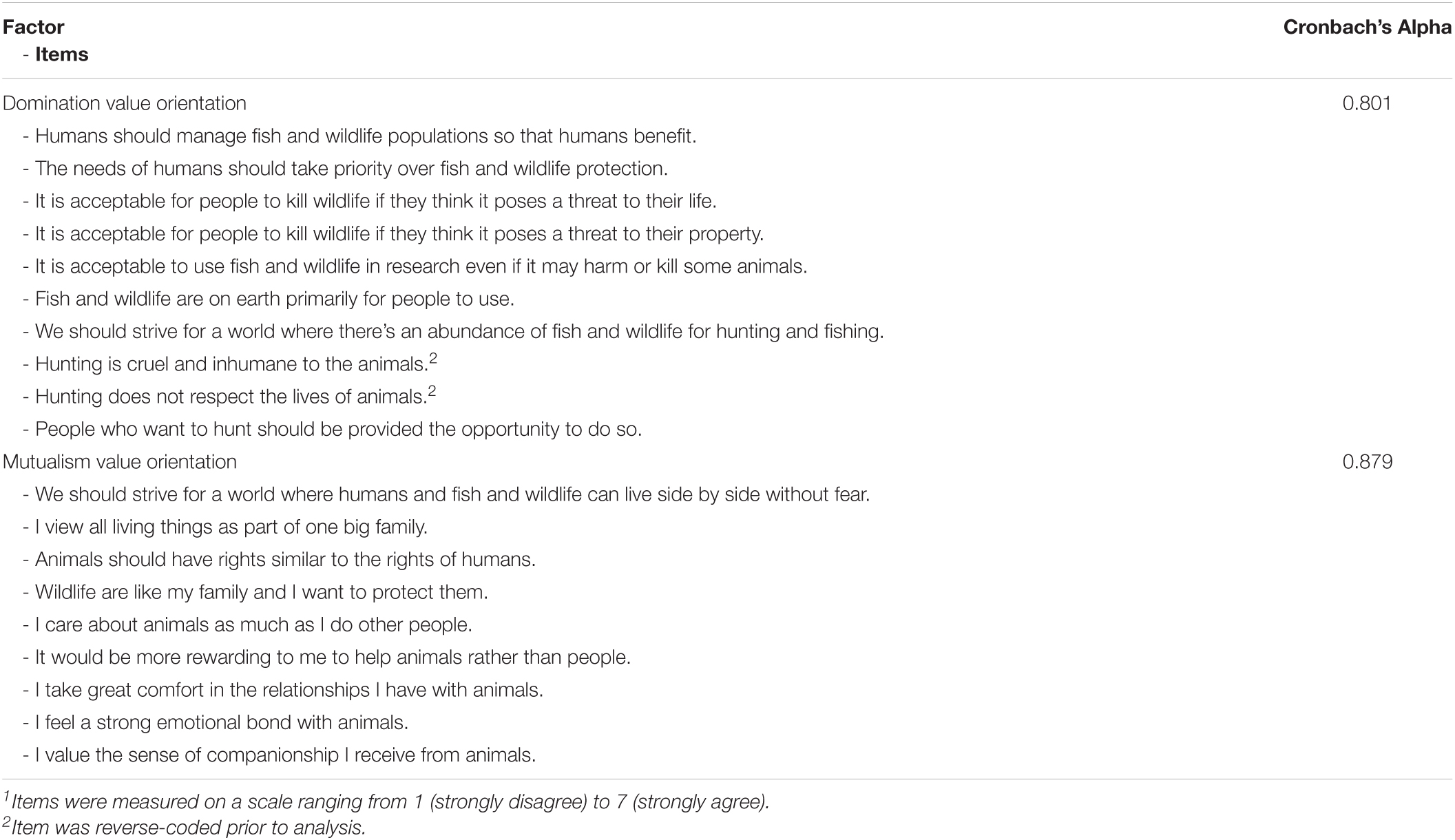In the upper left corner of the image, the text reads "Factor Items," followed by "Factor" and "Items" below it, separated by a line. On the right side, the text reads "Cronbach's α" with a line underneath it. Both these sections are enclosed by light gray lines above and below them. Underneath these headings, the text "Domination Value Orientation" appears.

The content is formatted with bullet points, represented by small dashes. The bullet points include the following statements:

- "Humans should manage fish and wildlife populations so that humans benefit."
- "The needs of humans should take priority over fish and wildlife protection."
- "It is acceptable for people to kill wildlife if they think it poses a threat to their life."
- "It is acceptable for people to kill wildlife if they think it poses a threat to their property."
- "It is acceptable to use fish and wildlife in research even if it may harm or kill some animals."
- "Fish and wildlife are on earth primarily for people to use."
- "We should strive for a world where there is an abundance of fish and wildlife for hunting and fishing."
- "Hunting is cruel and inhumane to the animals" (accompanied by a footnote marker, “2”).
- "Hunting does not respect the lives of animals" (accompanied by a footnote marker, “2”).
- "People who want to hunt should be provided the opportunity to do so."

Following these points, the text "Mutualism Value Orientation" appears, indicating a shift in the thematic category of the items listed.